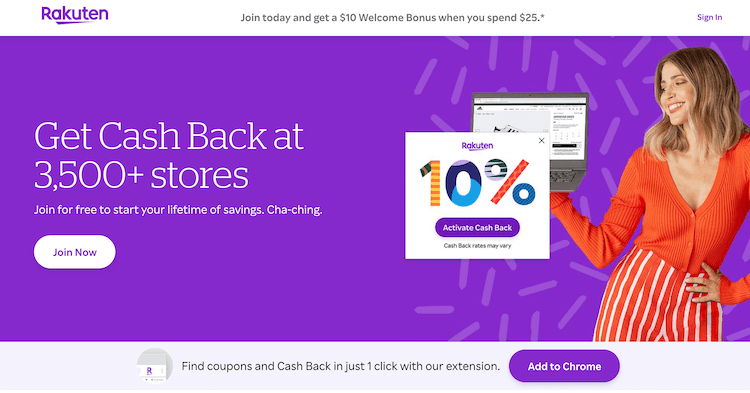This image is a screenshot of an advertisement for a website named "RAKULIN." At the top left corner, there is a white navigation bar featuring the website's name "RAKULIN," with the letters "K" and "U" underlined by a dash. Adjacent to this, in a grey font, the text reads, "Join today and get a $10 welcome bonus when you spend $25*," with an asterisk indicating some conditions apply. Positioned in the upper right corner, the option to "Sign In" is displayed in blue font.

The advertisement itself has a vibrant purple background. On the right side of the ad, there is an image of a woman with shoulder-length blonde hair, wearing a red sweater and red and white striped pants. She is smiling broadly at a laptop that appears to be photoshopped into her hand. Overlaying the laptop is a white square featuring the "RAKULIN" logo, a "10% off" promotion, and the message "Activate cashback. Cashback rates may vary."

To the left of the woman, in a solid purple section, white text encourages users to "Get cashback at 3,500+ stores. Join for free to start your lifetime of savings." At the bottom of this motivational message, the phrase "Cha-ching!" adds a playful touch, suggesting the financial benefits of joining the website.